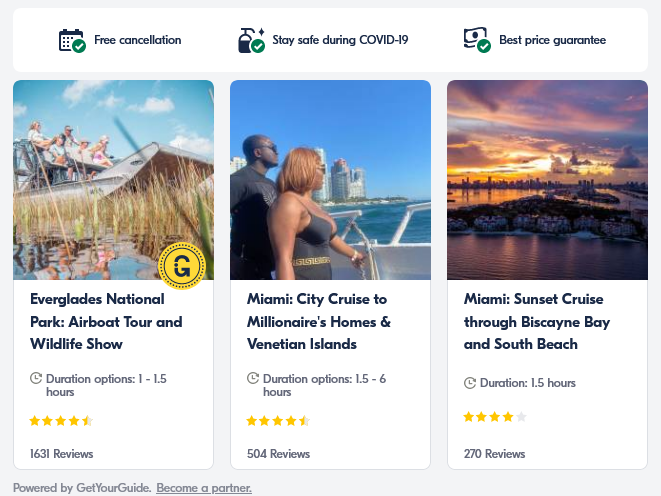The image is a screen capture featuring a white background showcasing a series of travel-related listings. At the top, in black font, there is a section highlighting key features, each accompanied by a green circle with a white check mark. The first feature reads "Free Cancellation" with a calendar icon. The second says "Stay Safe During COVID-19" featuring a pump bottle with soap icon. The third states "Best Price Guarantee" alongside a dollar bill icon.

Below these features is a listing for the "Everglades National Park Airboat Tour and Wildlife Show." The tour duration is between one to one and a half hours and it has received an average rating of 4.5 stars from 1,631 reviews. The listing is powered by GetYourGuide, indicated by a gold circle with a navy "G." The accompanying image shows a family on an airboat in a marsh, surrounded by plant life.

Next is the listing for the "Miami City Cruise to Millionaire's Homes in Venetian Islands." The tour duration ranges from one and a half to six hours, with a rating of 4.5 stars from 504 reviews. The image depicts an African-American couple enjoying the turquoise water with high rises in the background under a blue sky.

The final listing is for the "Miami Sunset Cruise through Biscayne Bay and South Beach." This tour lasts 1.5 hours and is rated 4 stars based on 270 reviews. The image shows a stunning sunset with vibrant purple, blue, orange, and yellow clouds, high rises and skyscrapers in the distance, and a body of water with waterfront homes.

This image neatly organizes travel options with informative and appealing visuals, offering a comprehensive overview of exciting tour choices.